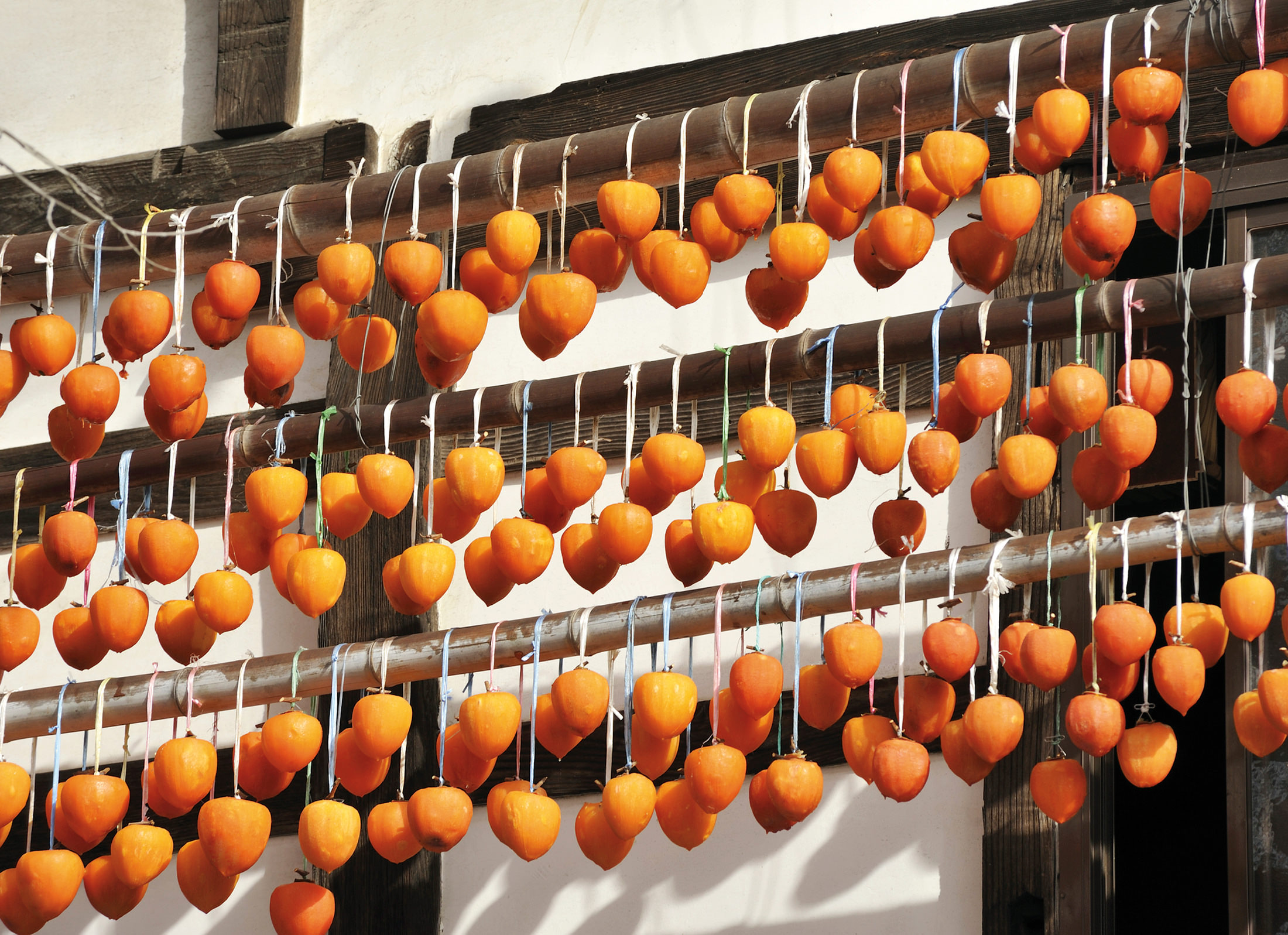The image depicts the outside of a rustic whitewashed building with dark wooden beams crisscrossing its facade. Prominently featured are three brown wooden rafters extending horizontally. Hanging from these rafters by white strings are dozens of slightly tear-shaped, orange-colored fruits, possibly persimmons, oranges, or apricots. Each string appears to hold two fruits, looped over the rafters. The fruits, likely intended for drying or sale, add a vibrant pop of color against the white and wooden background. In the mid to bottom right-hand corner, a door or window pane is faintly visible. The scene captures an intriguing blend of traditional agricultural practice and rustic architecture.